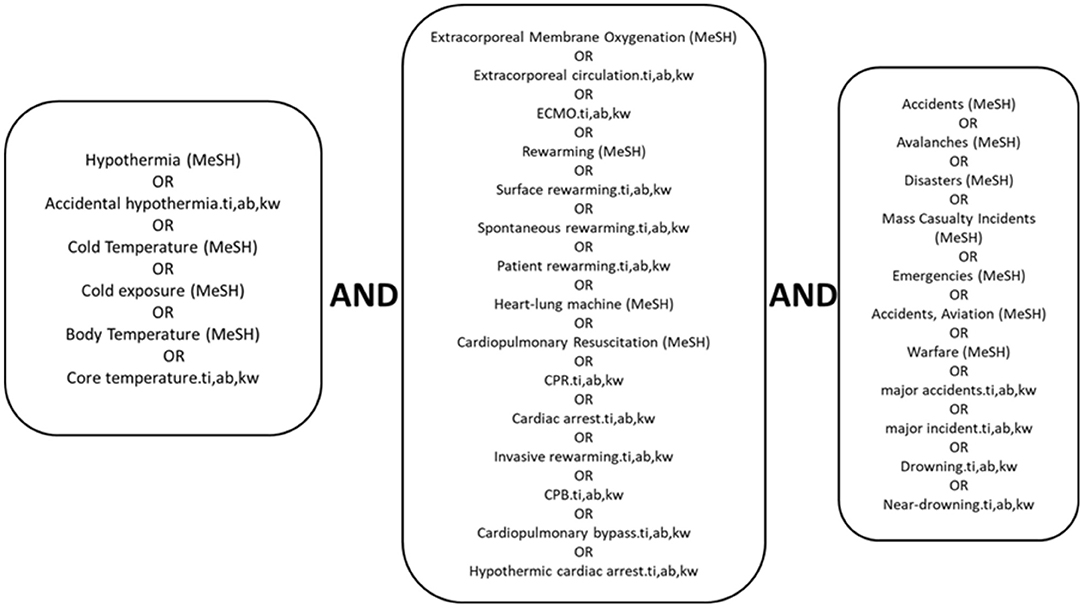The image is a detailed, black-and-white diagram divided into three distinct vertical columns separated by the word "AND" in bold text, resembling something from a scientific textbook. The first column, squarish in shape, lists terms like hypothermia, accidental hypothermia, cold temperature, cold exposure, body temperature, and core temperature. The second, more rectangular and longer column includes terms such as extracorporeal membrane oxygenation (ECMO), extracorporeal circulation, rewarming, surface rewarming, spontaneous rewarming, patient rewarming, heart-lung machine, cardiopulmonary resuscitation (CPR), cardiac arrest, invasive rewarming, cardiopulmonary bypass (CPB), and hypothermic cardiac arrest. The third, narrower and shorter column, covers terms related to accidents or avalanches, disasters, mass casualty incidents, emergencies, aviation accidents, welfare, major accidents, major incidents, drowning, and near drowning. Overall, it's a comprehensive diagrammatic representation with logical operators 'OR' and 'AND' linking medical and emergency terms associated with hypothermia and related treatments and situations.